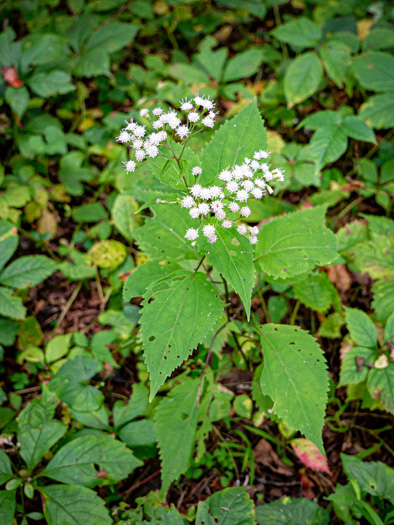The photograph displays a rectangular image, twice as long as it is tall, with a flower centered precisely in the frame. This flower comprises multiple small, many-petaled white blossoms featuring yellow dot-like centers, each sprouting from slender green stems. These stems converge onto thicker, brown stems, forming two clumps part of a Y-shaped structure. Accompanying the flowers are large, teardrop-shaped leaves with visible ridges; many of these leaves bear holes likely caused by insects or other creatures. The setting is a brown, vegetated floor interspersed with twigs and scattered foliage. Surrounding the central plant, additional green leaves, some imperfect due to bug predation, and various smaller plants such as four-leaf clovers and poison ivy contribute to the natural, somewhat untamed atmosphere. Small red buds add a subtle dash of color among the predominantly green scenery.